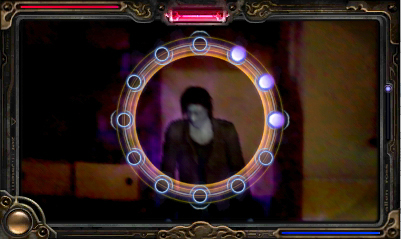The image is a still from a video game, captured horizontally, and it is encased in a frame that appears to be crafted from gilded metal. The ornate detailing around the edges of the frame lends it a luxurious, almost antique appearance. At the bottom left corner of the frame, a prominent golden circle catches the eye. The top section of the frame features a distinct red area, presumably for indicating the player's health status.

In the center of this framed scene stands the player character, clad in sleek black attire, their gaze cast downward, evoking a sense of contemplation or readiness. Encircling the character is an intricate ring, marked by several smaller circles. Notably, three of these circles within the ring are illuminated, suggesting they are activated or hold special significance in the game's context. The detailed imagery and design elements combine to create a rich, immersive visual experience.